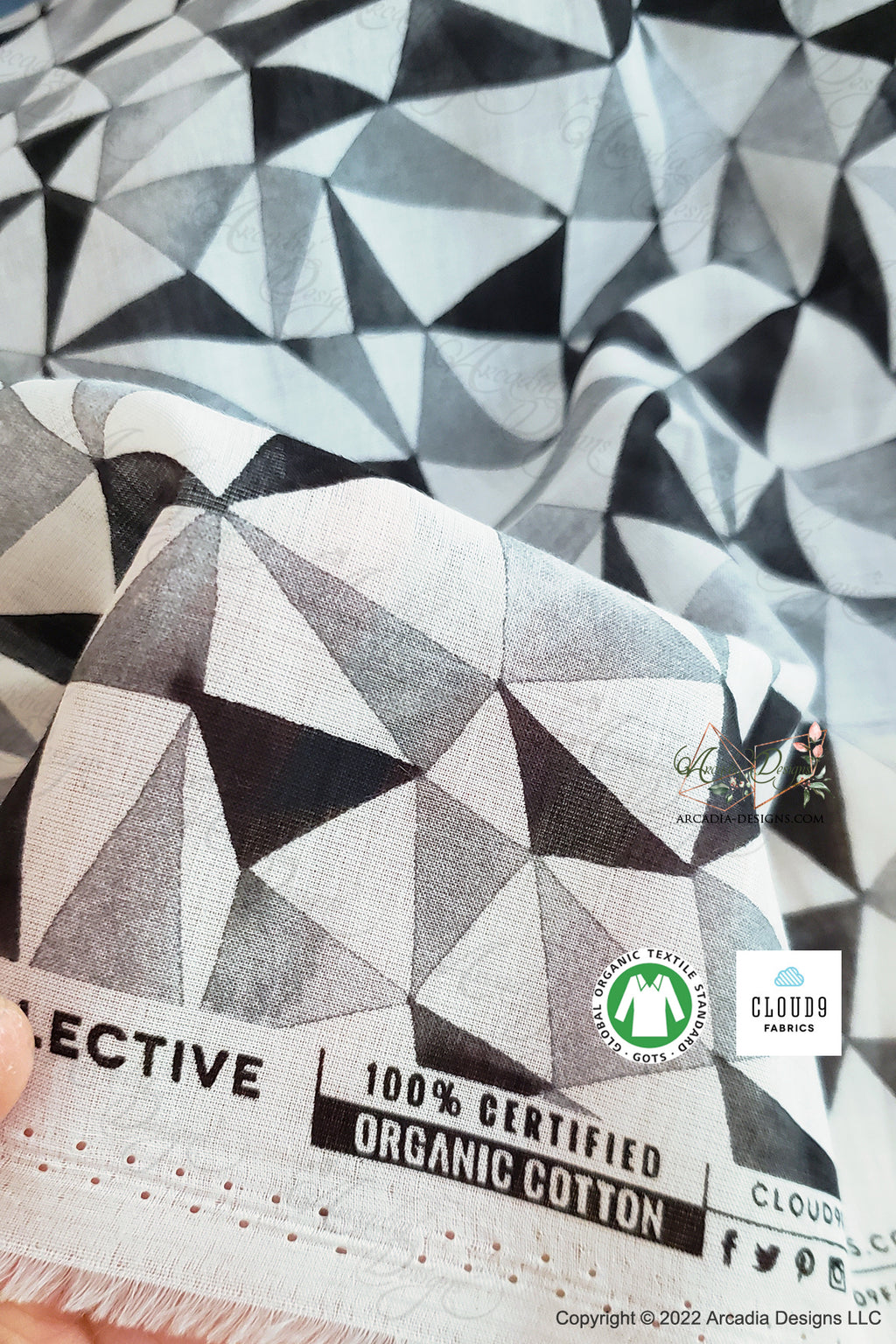This detailed photo showcases a piece of fabric adorned with a pattern of black, white, and gray triangles. The fabric is made from 100% certified organic cotton, as indicated by a visible tag. The texture of the fabric appears fine-grained and slightly crumpled, with some fringe visible at the bottom edge of the image. 

The fabric also features several tags: a rectangular tag with the words "Cloud 9 Fabrics" and an Organic Textile Standard logo, which includes a green circle displaying a white blouse, helping to identify the material. There is also a partially obscured tag with the letters "-E-C-T-I-V-E" visible, and a thumb covers part of this tag. 

Despite being slightly folded and without visible sleeves, the pattern and tags strongly suggest that this fabric is part of a larger garment, likely a blouse. The photograph captures the intricate details of the design and the material quality, emphasizing its organic and certified nature.